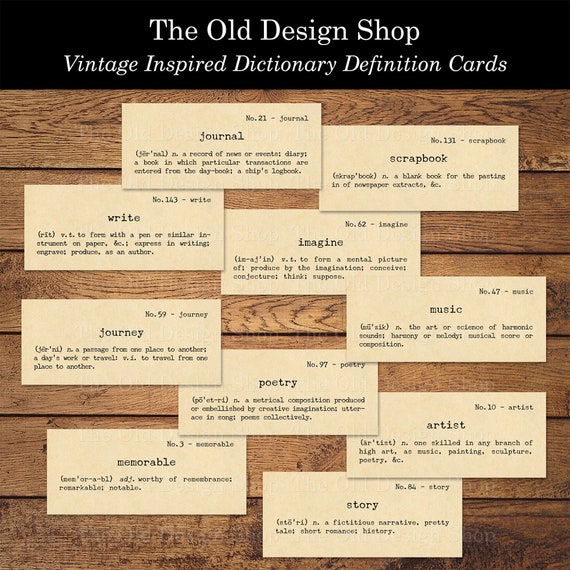This image appears to be an advertising or product photograph for vintage-inspired dictionary definition cards. At the top of the image, the text reads "The Old Design Shop." The cards are described as "Vintage-Inspired Dictionary Definition Cards." The cards are displayed in a neatly stacked pile on a rustic wooden background, enhancing the vintage aesthetic. Each card features a word along with its definition. The visible card highlights words such as "journal," "scrapbook," "music," "journey," "poetry," "artist," "memorable," and "story," each accompanied by their respective definitions. This setting suggests a creative environment, ideal for art, journaling, and storytelling.